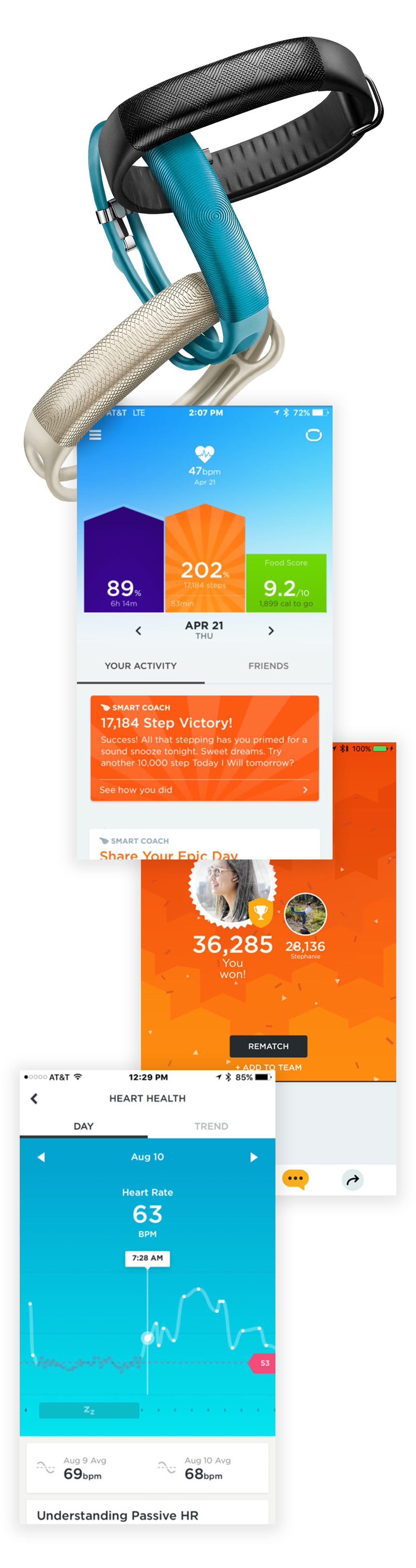The image is an advertisement for a fitness monitoring product. At the top of the tall photograph, three wristbands are connected in a descending chain, forming a visually appealing bracelet stack. The top band, which is black and leather-like, leans towards the upper right corner. Connected to it is a blue band, angled from left to right. The final band is off-white, connecting diagonally from the right down to the left.

Hanging from these bands are various rectangular inserts that resemble screenshots from a smartphone. The layout seems to include a black circular band at the top, from which blue and silver carabiners dangle, holding numerous images.

The top image features text that reads, "Your Activity, April 21st, Thursday." It mentions a "Smart Coach" with a "17,184 Step Victory, Success," and motivational messages like "All that stepping has you primed for a sound snooze tonight. Sweet Dreams," urging users to aim for "Another 10,000 Step."

The next image showcases a color photograph of a woman facing left, accompanied by the text "36,285, You Won!" Below this is another color photograph with a not-so-clear image, labeled "28,136, Stephanie."

Further down, another insert focuses on heart health, reading "Heart Health, August 10th, Heart Rate 63 BPM, 7:28 AM. August 9th, Average 69 BPM. August 10th, Average 68 BPM, Understanding Passive HR."

Collectively, these inserts, highlighted by the attached bands, detail various fitness metrics, achievements, and heart health readings, suggesting a comprehensive fitness tracking system.